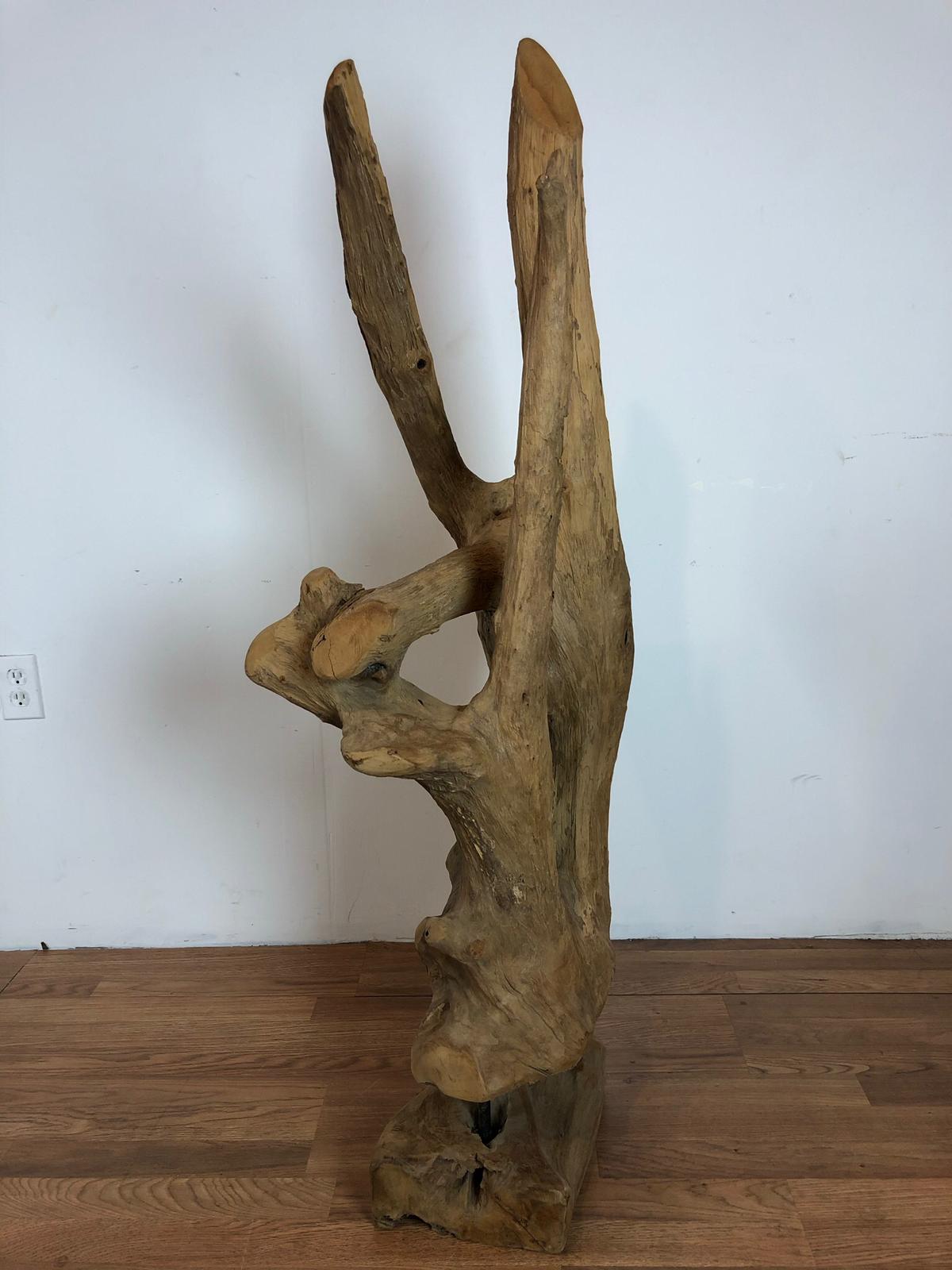This indoor photograph features a striking piece of driftwood, expertly transformed into an artful sculpture. The driftwood, positioned on a dark brown hardwood floor, has a rich, medium-brown hue that's slightly lighter than the floor itself. The stark contrast is accentuated by the pristine white wall in the background. The natural form of the driftwood vaguely resembles a hand, with two 'fingers' branching upwards and another one curving down to touch a side branch, mimicking the touch of a thumb and ring finger. The base of the driftwood appears to be meticulously trimmed and carved into a stable, rectangular shape, ensuring it stands upright, while the rest of the structure retains its organic character, weathered by time. Notably, the tip on the right side looks particularly smooth as if it has been cut. The piece also displays an array of browns – from lighter tones to darker patches – enhancing its textural complexity and visual appeal. This artistic display of natural beauty captures the eye, embodying both craftsmanship and the raw elegance of nature.